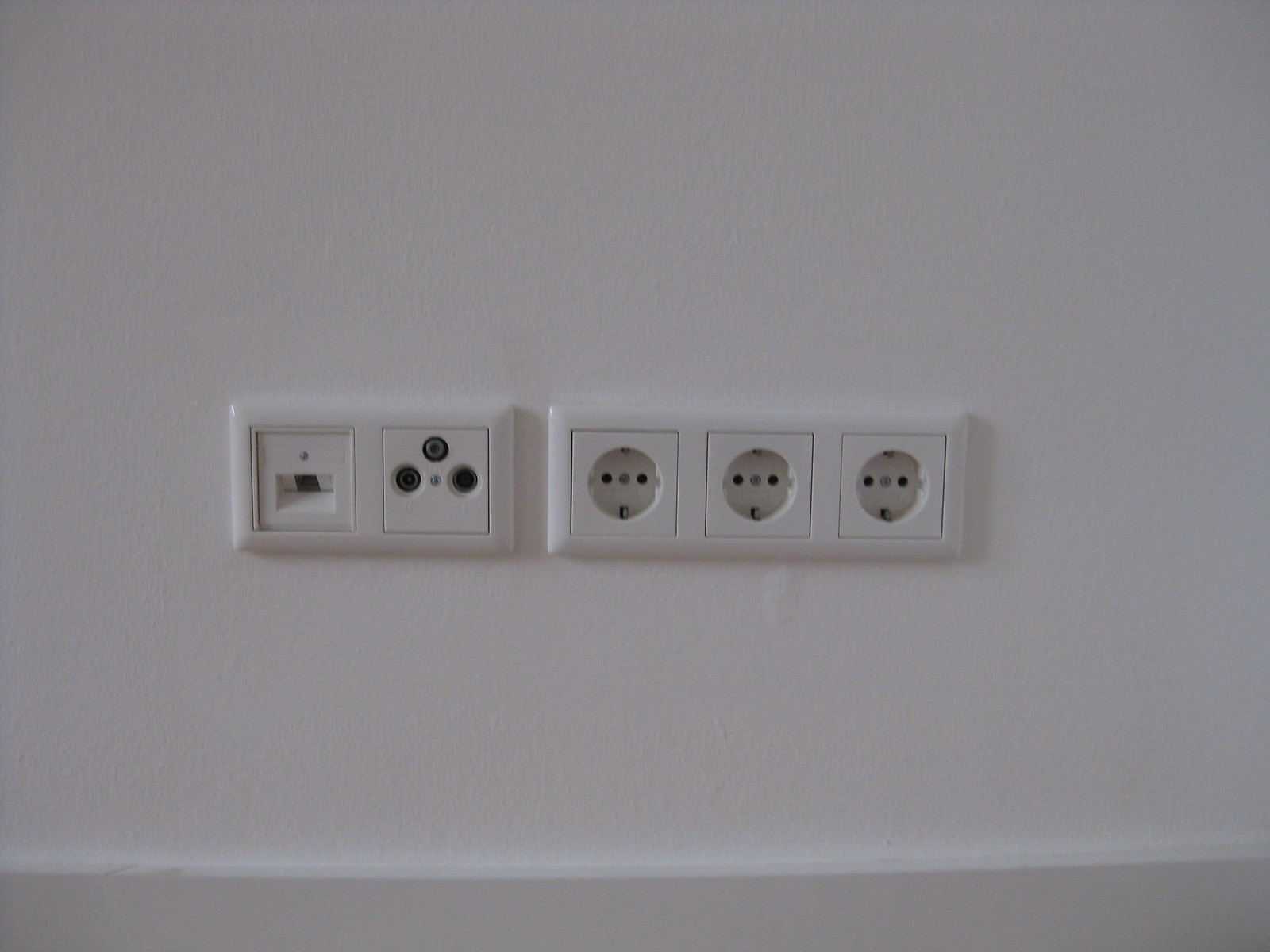The image features a zoomed-in view of a plain white wall, showcasing five distinct electrical outlets. The bottom part of the wall includes a white baseboard with some gray scuff marks on the left side. The outlets are arranged in two groups, one of two and one of three, each housed within its own outlined square. The group of three outlets on the right appears to be European style, featuring three prong holes in a vertical alignment with an additional prong hole directly below them. The set of two outlets on the left includes one with a single square opening and another with three circular openings, one of which has a silver dot in the center, possibly indicating a specialized connector. These unique sockets suggest European or possibly Asian electrical standards, with one outlet potentially being a phone jack.